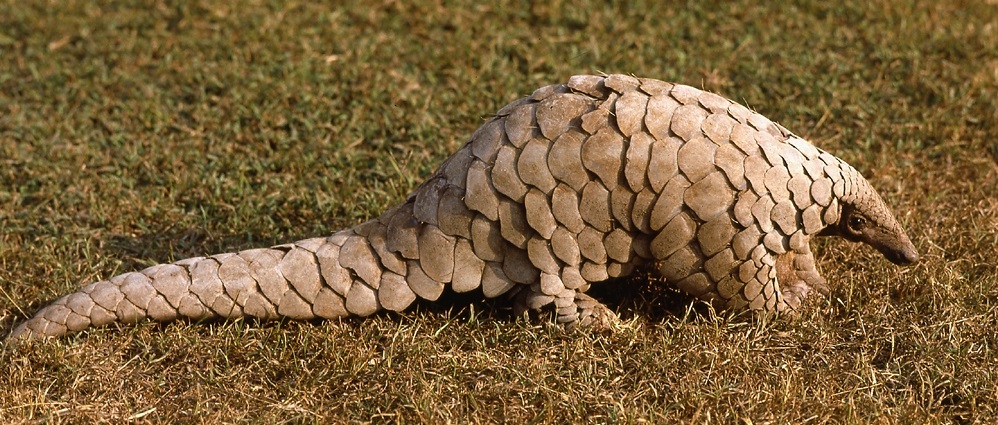The image captures a pangolin in detailed profile, standing outdoors on a field of grass during the daytime. The pangolin, with its light gray-brown scales reminiscent of dragon armor, occupies nearly the entire frame from its small, elongated head with a black snout to its lengthy tail stretching to the far left. Each overlapping scale contrasts in size, becoming smaller near the face and larger towards the back. The grass beneath the pangolin varies in color and clarity, transitioning from a sharper, drier brown in the foreground to a blurrier, vibrant green in the background, indicating a well-lit, sunny day. Every plate on the pangolin's body is distinctly visible, highlighting the textured armor-like appearance.